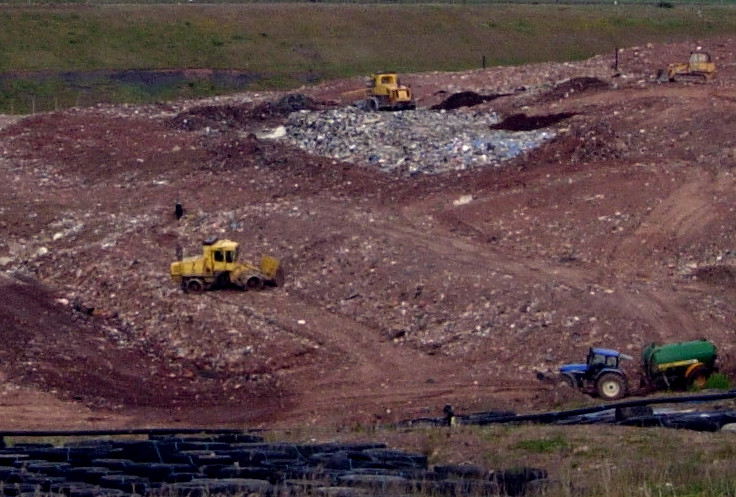The image depicts a sprawling landfill site characterized by predominantly red-brown dirt. At the center and middle left of the image, you can see heavy-duty yellow construction vehicles, possibly bulldozers, actively working on the site. Another yellow vehicle is positioned towards the top middle, navigating a grayish circular patch amidst the otherwise red-brown terrain. The right side of the scene features a small yellow bulldozer and, in the front right corner, a little blue tractor pulling a green tank, which gives an almost toy-like appearance due to the apparent distance from which the photo was taken.

Scattered across the landfill are mounds of white and gray rubbish, adding to the chaotic yet industrious atmosphere. In the distant background, a grassy hill rises, adorned with verdant grass and sporadic trees, contrasting sharply with the desolate, cleared area of the landfill. The entire scene captures the dynamic interplay between industrial activity and the remnants of natural scenery.